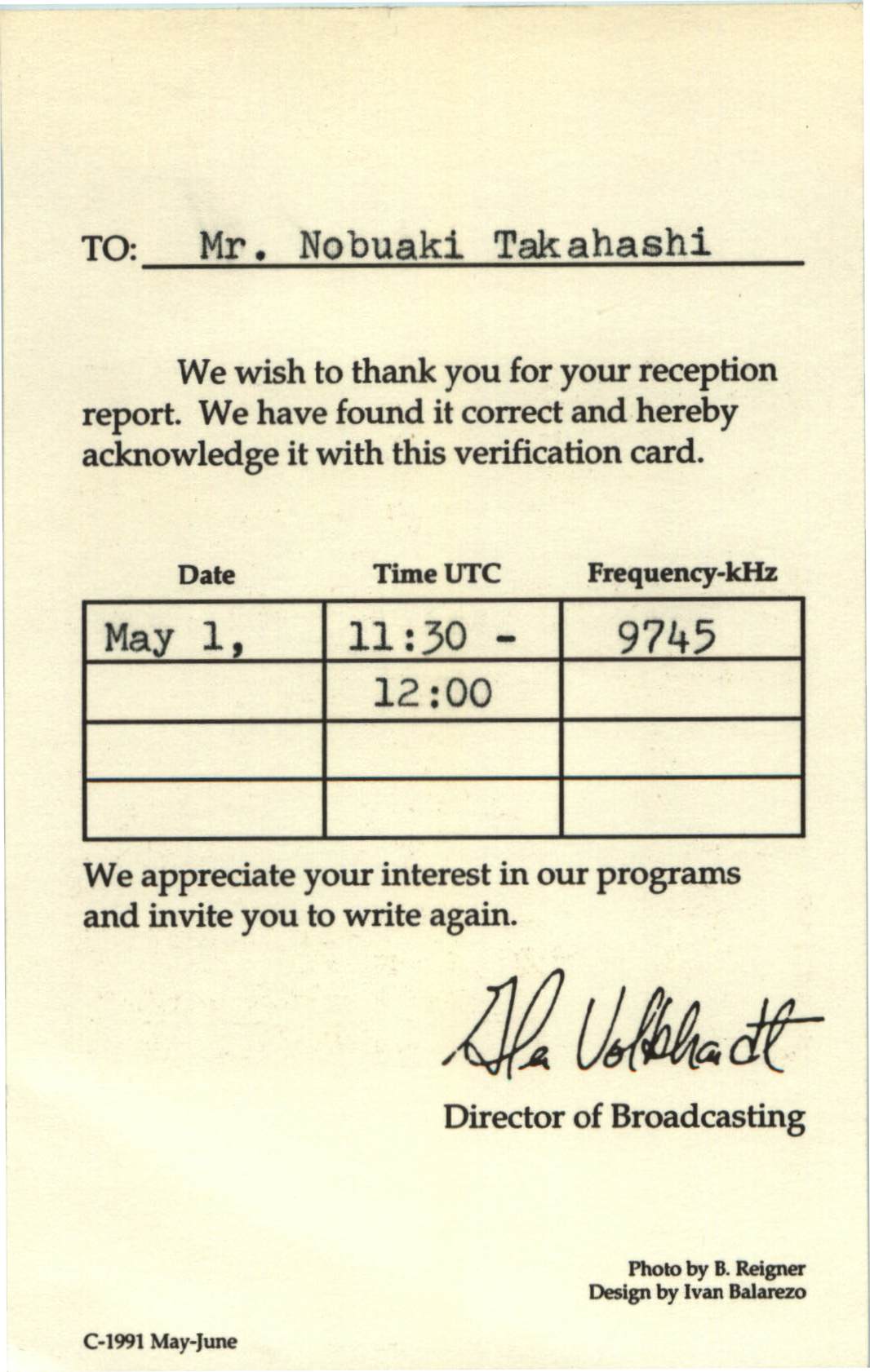The image depicts a yellow verification card addressed to Mr. Nobuaki Takahashi. The top of the card reads, "We wish to thank you for your reception report. We have found it correct and hereby acknowledge it with this verification card." Below is a table with the following details: Date - May 1st, Time (UTC) - 1130 to 1200, and Frequency - 9745 kHz. Underneath the table, the card states, "We appreciate your interest in our programs and invite you to write again." The card is signed by an illegible signature denoting the Director of Broadcasting. The bottom right corner notes "Photo by B. Rainer, designed by Ivan Balarezo," while the bottom left-hand corner includes "C-1991, May-June."